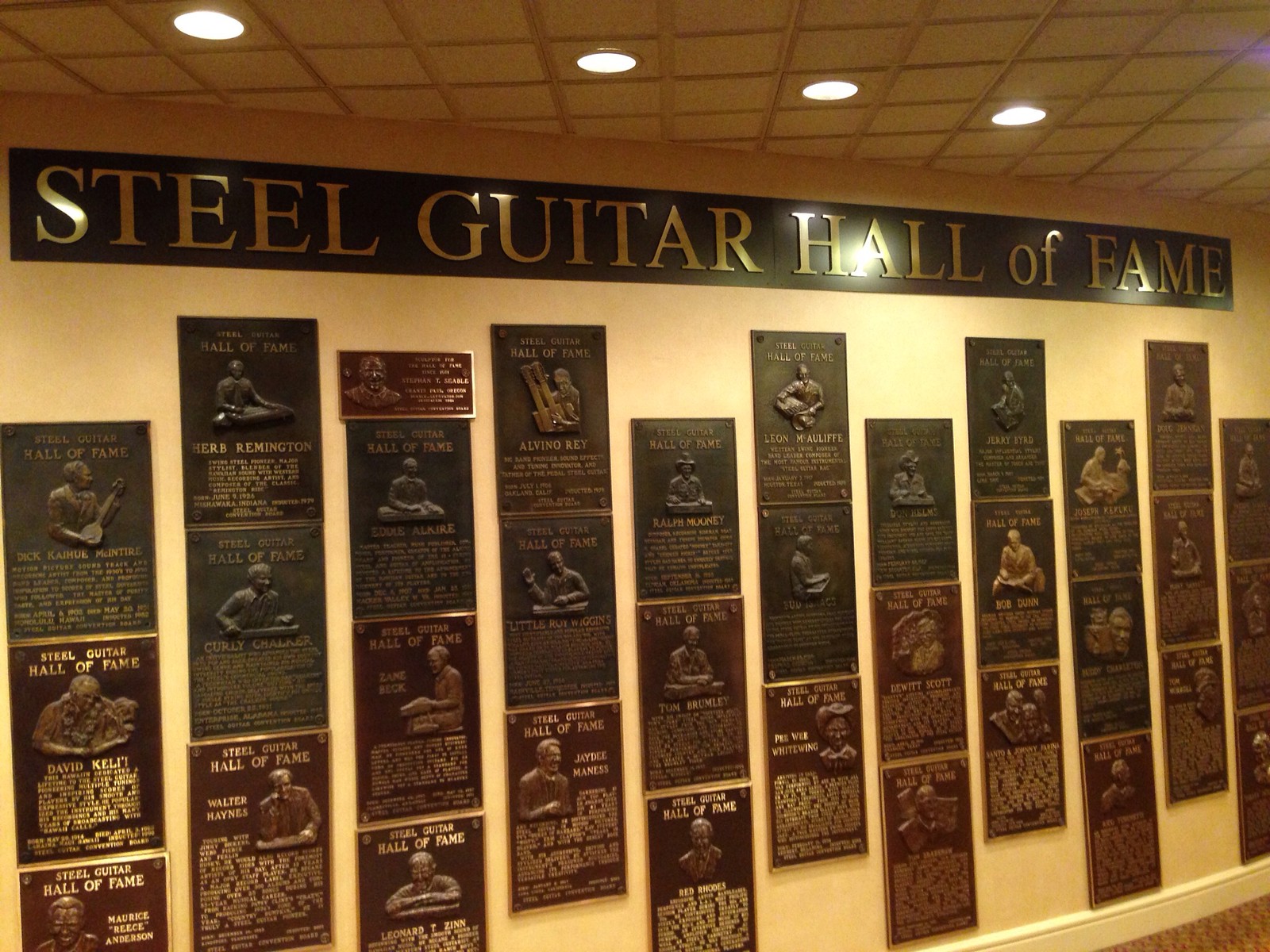The photograph depicts a room with light yellow walls and matching light yellow molding, partially revealing a corner of brown carpet. The ceiling is adorned with brown tiles and a row of small lights. Dominating the wall is a long black frame with gold 3D letters that spell out "STEEL GUITAR HALL OF FAME." Below this bold title, arranged neatly in about a dozen columns, are bronze plaques, each featuring an artist's image and name, alongside smaller text that is too small to read. This display honors various individuals inducted into the Steel Guitar Hall of Fame.